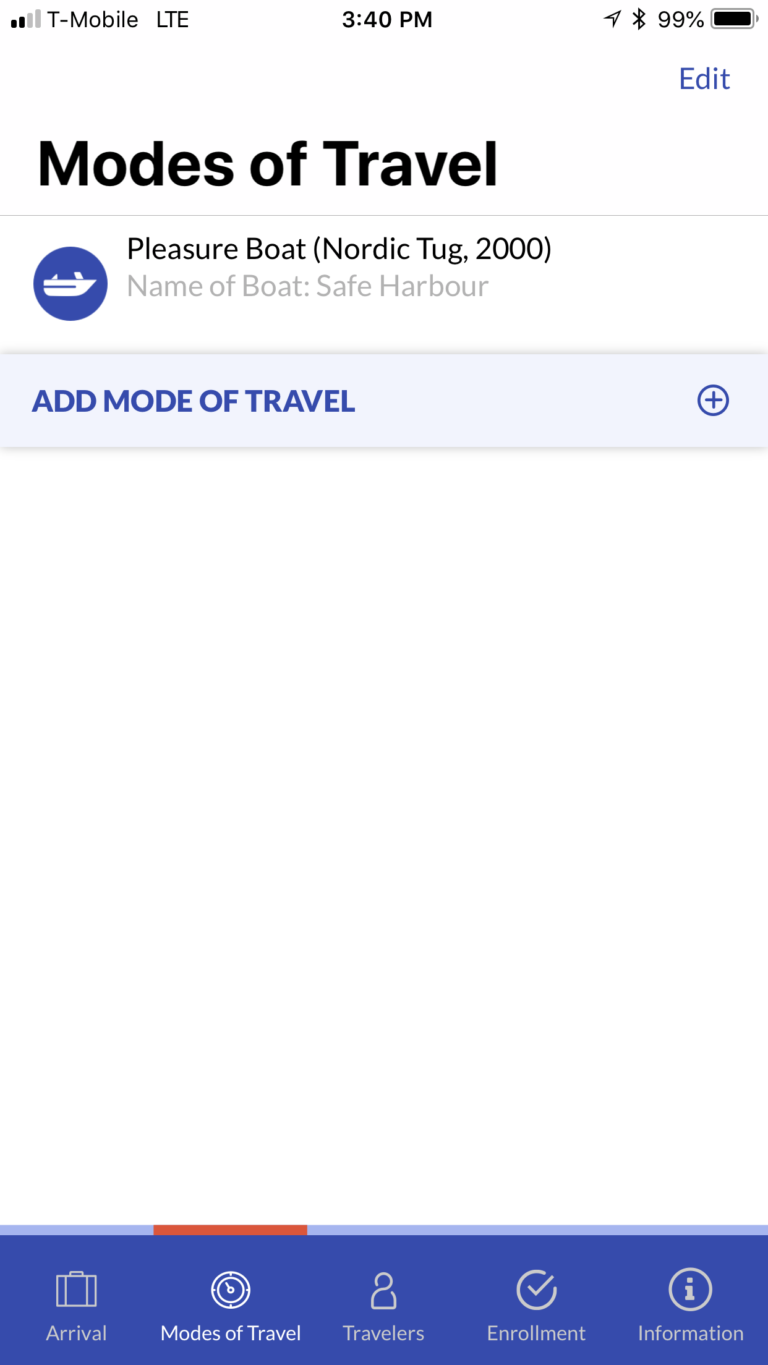Screenshot of a Mobile Travel App Interface:

This screenshot captures the user interface of a predominantly white-themed travel app. At the top left corner, in large bold black letters, is the heading "Modes of Travel." Directly beneath this title, there is a section showcasing various transportation methods. 

The first item in this section features a boat icon followed by the text "Pleasure Boat (Nordic Tug 2000)." Underneath this, in smaller grey letters, it specifies the boat's name, "Safe Harbor."

Below this information, a blue rectangular box is visible with the text "Add Mode of Travel" in light blue font. Just to the right of this box, aligned to the far edge of the page, is a plus icon that allows users to add another travel mode.

At the bottom of the screenshot, there is a navigation bar with five horizontally aligned icons:

1. A suitcase icon labeled "Arrival."
2. A compass icon labeled "Modes of Travel."
3. A person icon labeled "Travelers."
4. A checkmark icon labeled "Enrollment."
5. An eye icon labeled "Information."